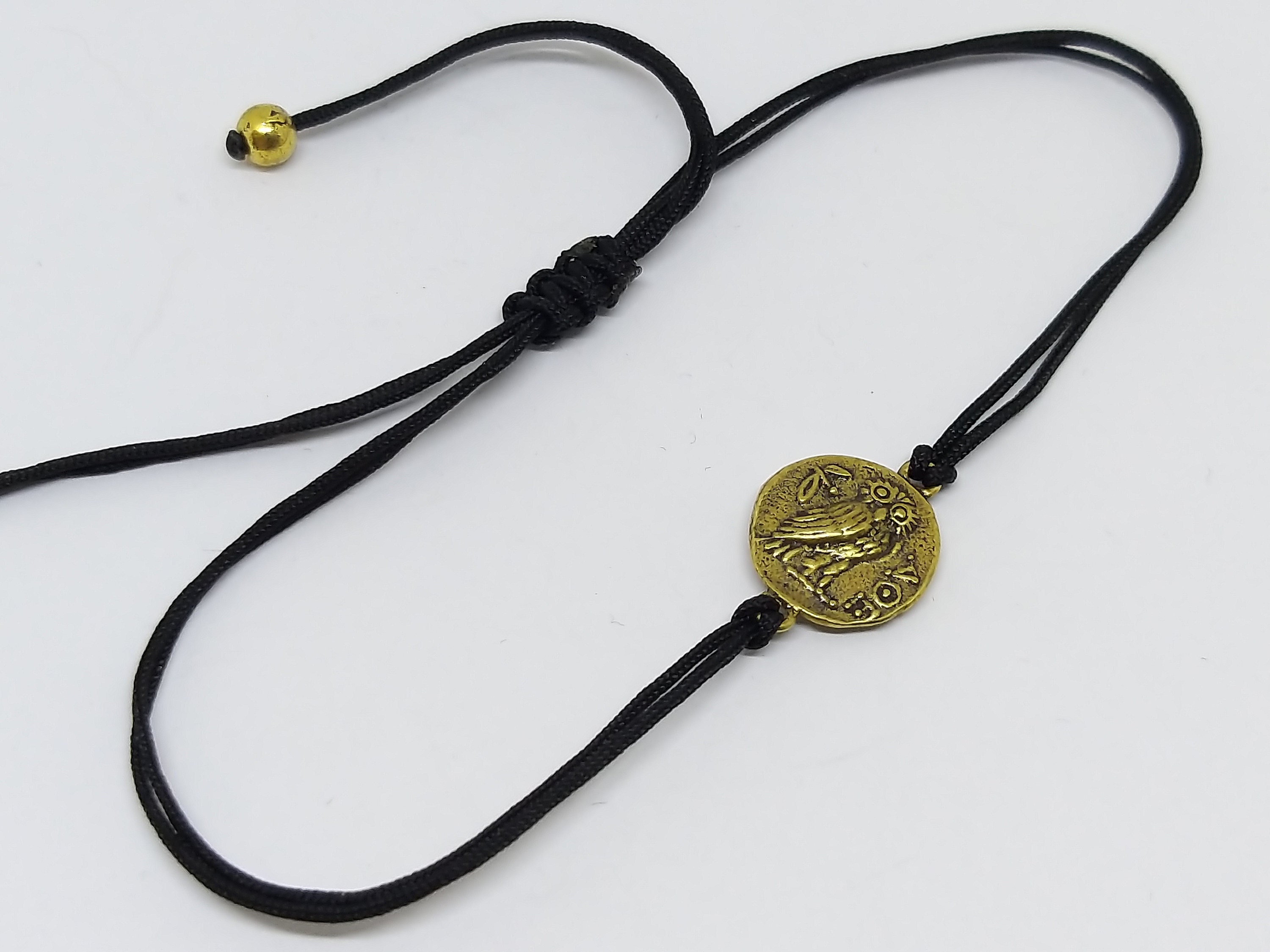In this image, we see a piece of jewelry that could function as both a choker necklace and a bracelet. It features a striking black cord that forms an oval shape when laid flat on a white tabletop. The cord is intricately tied in several loops at the back, with a pair of golden beads dangling from the loose ends, allowing for adjustable tightness.

Attached to the cord is a pendant resembling an antique coin, though it is not genuinely aged. This round, gold-colored coin sports a distinct patina, adding to its vintage allure. Dominating the coin's design is a rudimentary depiction of an owl, facing right with its body while its head gazes forward. The owl's large, circular eyes and visible wing contribute to its tramp art style, which is not heavily detailed. Near the owl, there are Greek letters inscribed, appearing as "A-O-E" or "V-O-E."

The coin is securely fastened to the cord with two gold loops, one at the top and one at the bottom. Overall, the piece exhibits a combination of rustic charm and classical elegance, suitable for various fashionable uses.